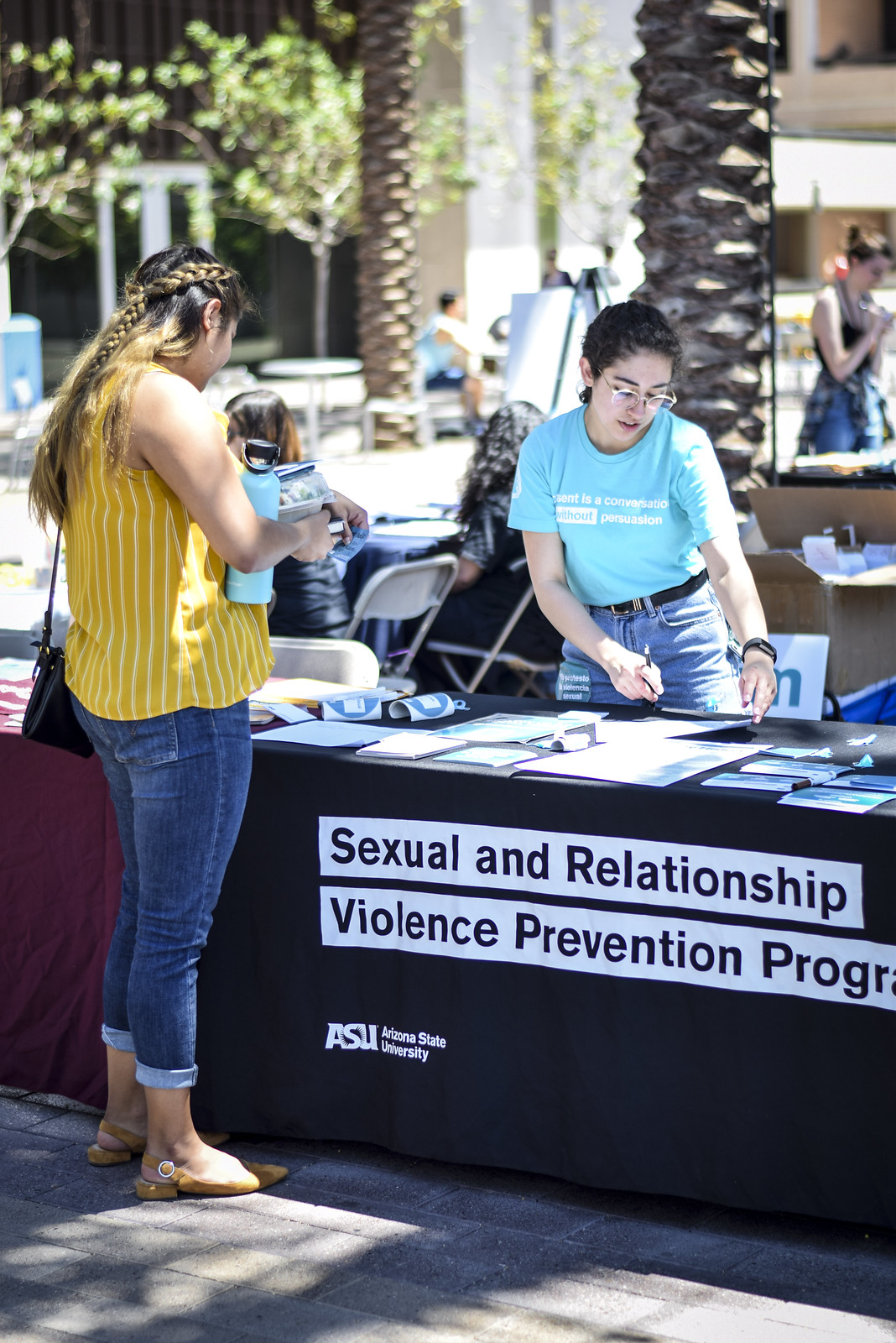In the image, there are several people outdoors, seemingly on a college campus, possibly an event at Arizona State University (ASU) focused on sexual and relationship violence prevention. A booth with a banner reading "Sexual and Relationship Violence Prevention Program" is prominently featured. On the left, a woman stands wearing a yellow and white striped tank top, blue jeans rolled up at the bottom, and orange shoes. She holds a light blue water bottle in her right hand and carries a black bag on her left shoulder. Her hair is braided. In front of her is a table with papers, appearing to provide information about the program. Behind the table sits another woman with black hair, wearing glasses and a blue short-sleeved t-shirt, accessorized with a black belt. She is looking down, possibly at the paperwork in front of her. The background reveals more booths, some trees, and other people walking around, albeit slightly blurred. The scene reflects a busy, engaged campus atmosphere dedicated to important social issues.